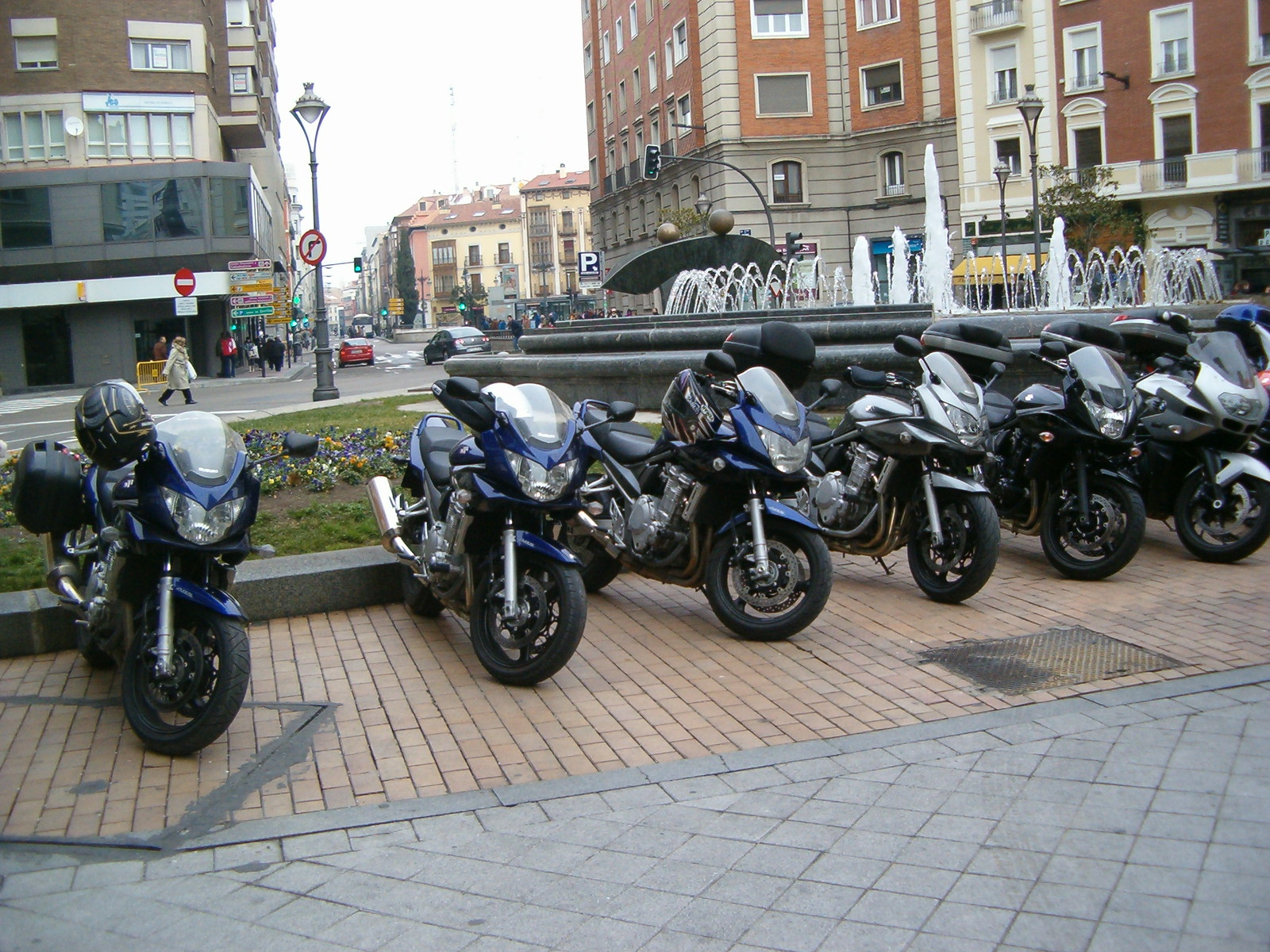The photograph captures a bustling city scene centered around a row of six motorcycles parked diagonally on a light brown or sandy-colored brick area. These motorcycles, facing the camera, display a mix of colors: the first three are a vivid blue with black seats and large wind guards, followed by a silver one, a black one, and another silver one. Directly in front of this bricked section lies a gray, diamond-patterned sidewalk. Behind the motorcycles, towards the right, stands a prominent round water fountain surrounded by a raised grassy bed adorned with flowers. The cityscape background reveals multi-story buildings, a mix of glass and brick exteriors, and bustling streets with a few pedestrians and cars. Notably, a tall building occupies the top left section of the image, featuring a glass center and brown and gray sections. A road stretches downward from the left side, adding depth to the urban atmosphere.